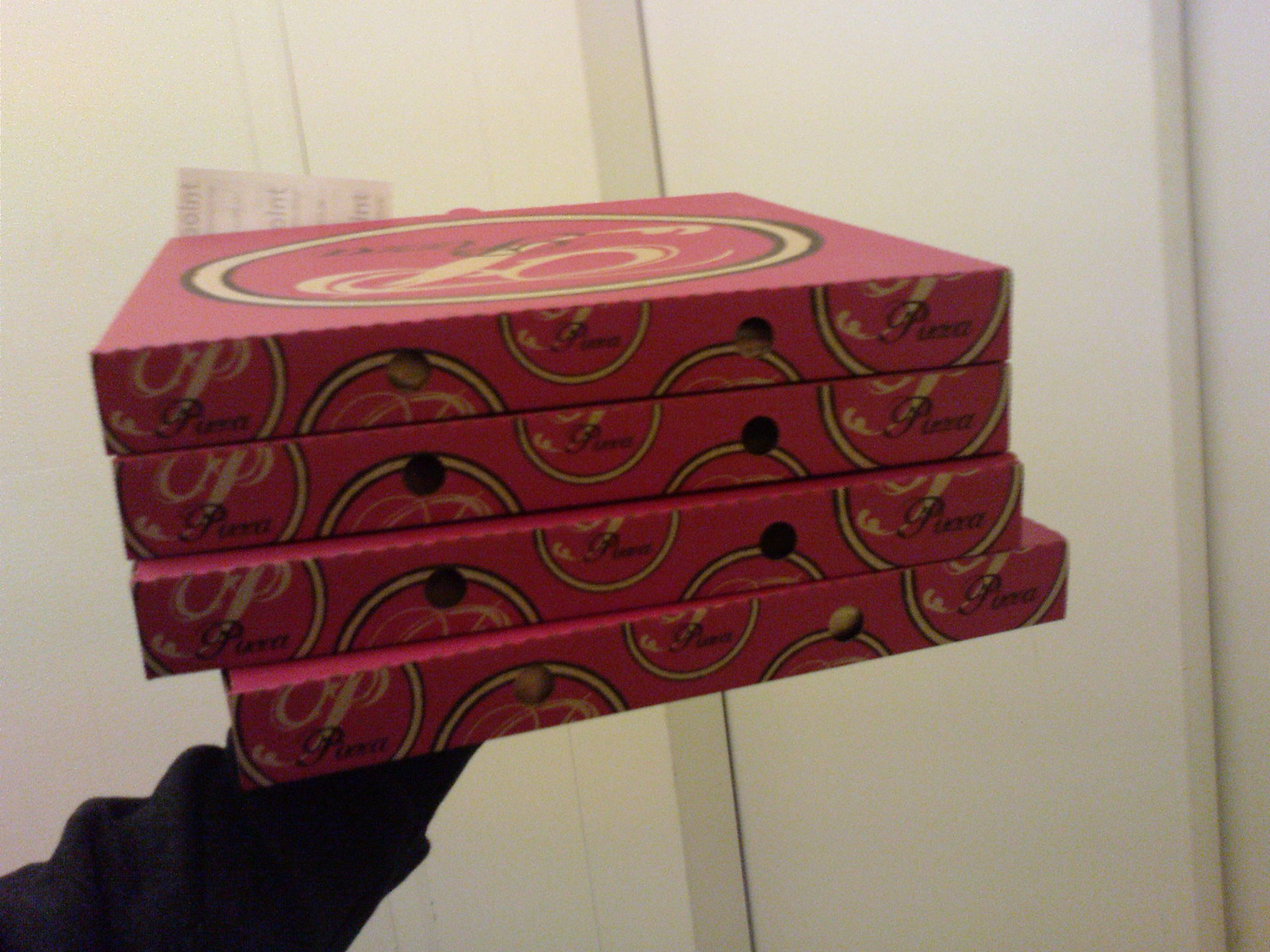A photograph taken indoors captures an arm in a black sleeve, presumably holding up four stacked, bright red pizza boxes. Each box features ventilation holes through which glimpses of the pizzas inside are visible. The boxes are emblazoned with consistent branding: a large yellow circle outlined in black is prominently displayed on the top, although the exact logo isn't fully discernible in the image. The sides of the boxes are decorated with black lettering that repeatedly spells out "pizza" and includes squiggly lines as part of the design. A receipt is visibly inserted into the top pizza box. The background is an off-white, paneled wall, contributing to the indoor and somewhat nondescript setting of the photograph.